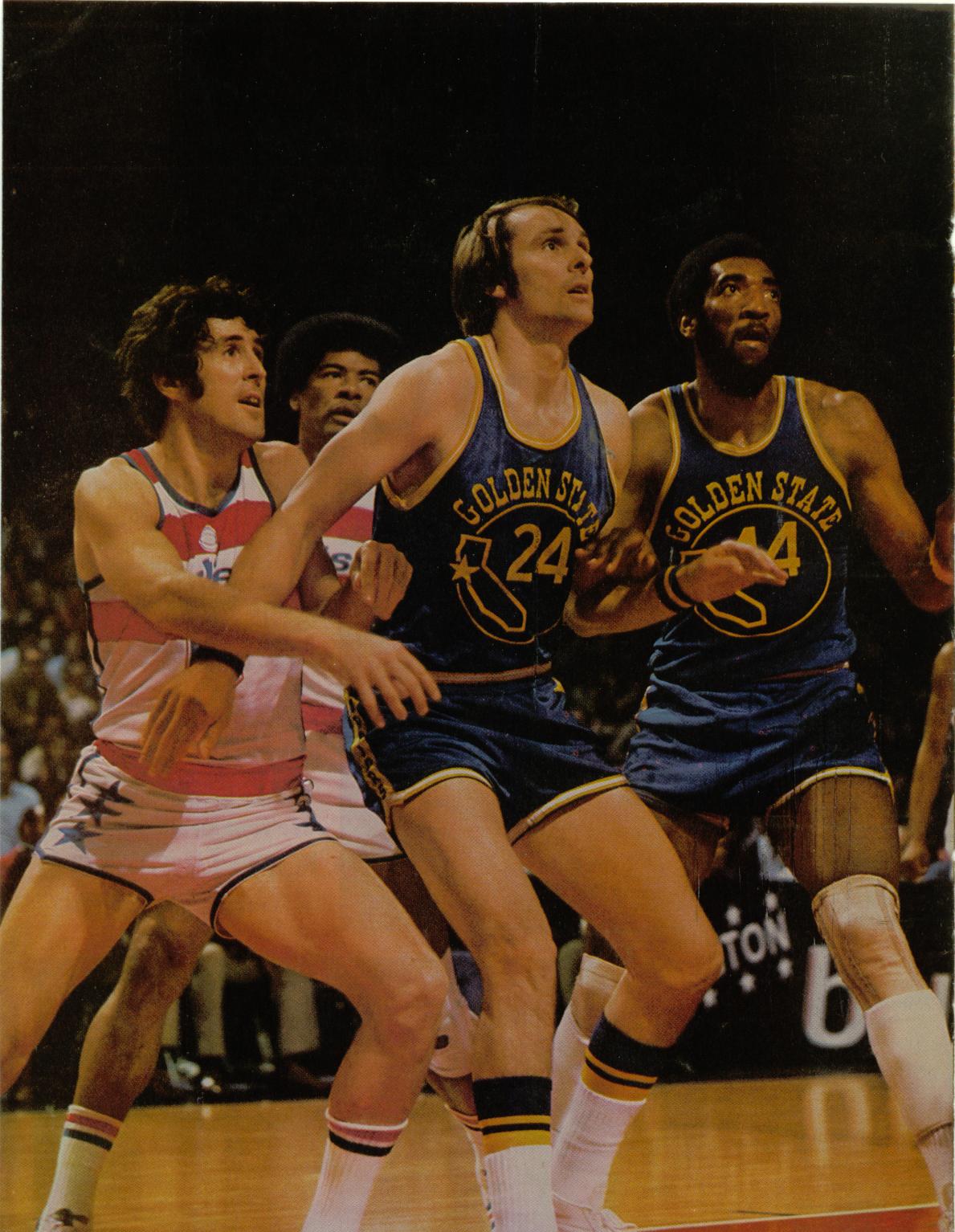The photograph captures a vibrant and nostalgic scene from a 1970s or 1980s basketball game. Centered on a polished light brown wooden basketball court, four male players from two opposing teams are the primary subjects, each dressed in distinct vintage uniforms. On the left, two players don red and white horizontally-striped sleeveless jerseys, paired with very short white shorts adorned with blue stars on the sides. On the right, the opposing team is clad in dark blue jerseys featuring yellow trim around the neck and arm openings, and matching yellow shorts with yellow stripes. The text “Golden State” is emblazoned on their jerseys, alongside illustrations of California and their numbers, such as 24 and 44. In the background, a blurred crowd fills the bleachers, intently watching the game. The overall setting is indoor, and the photo perfectly captures the vibrant colors and energy of a classic basketball match from this era.